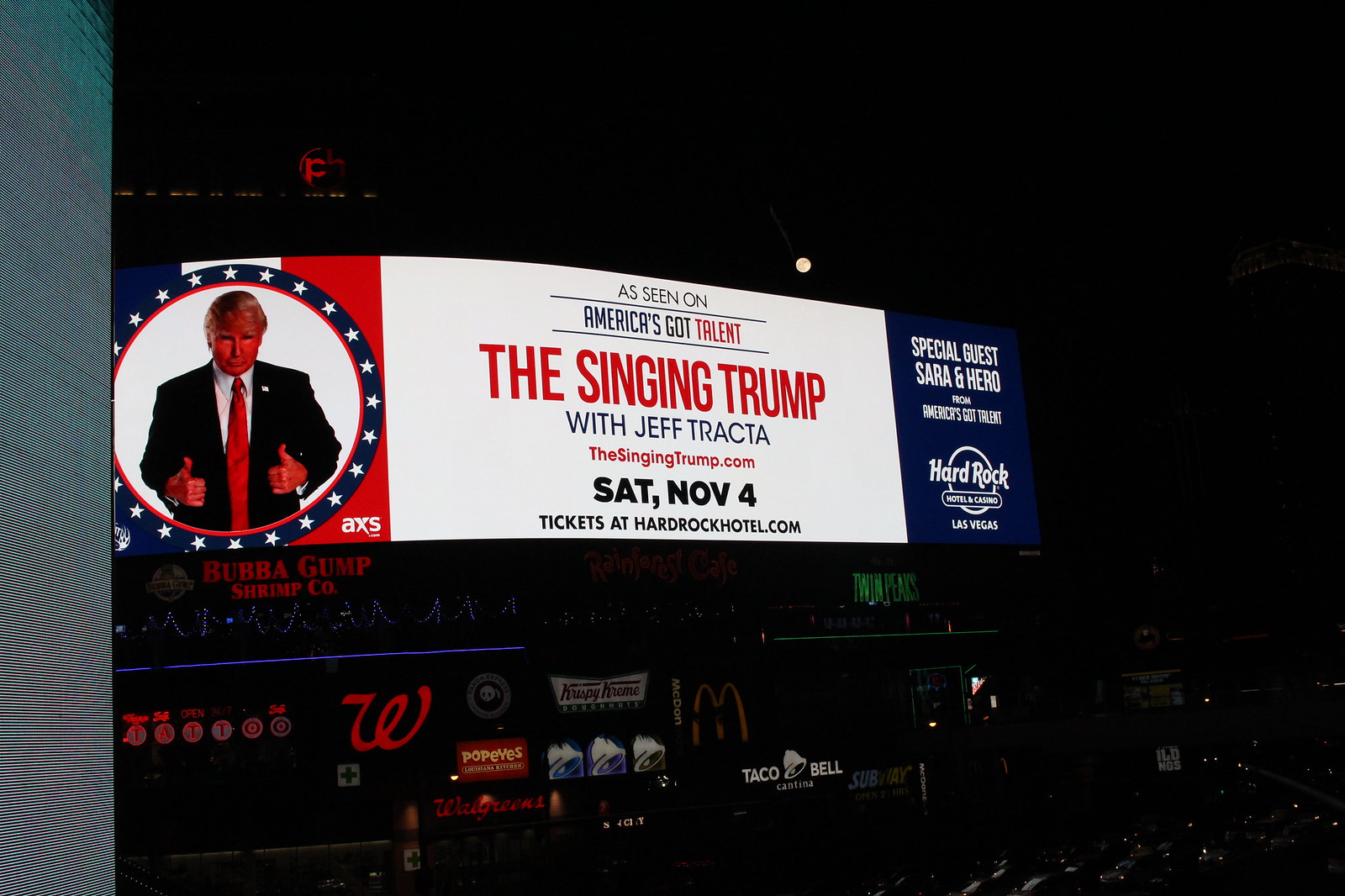The image features a large billboard-style advertisement attached to a building, designed to resemble an entertainment venue's promotional display. Dominating the left side of the billboard is a patriotic motif with red, white, and blue stripes accompanied by a circular blue area adorned with white stars, reminiscent of the American flag. At the center of the billboard, set against a white background, is an individual dressed as and resembling Donald Trump.

Prominently displayed in the white area of the sign are the words "A SCENE ON AMERICA'S GOT TALENT," followed by "THE SINGING TRUMP" written in bold red letters. Beneath this, in black letters, it reads "WITH JEFF TRAKTA," and further down in red letters again, "THE SINGING TRUMP DOT COM." The announcement continues in black text with "SATURDAY, NOVEMBER 4, TICKETS AT HARDROCKHOTEL DOT COM."

On the right-hand side of the billboard, set against a black background, the words "SPECIAL GUEST, SARAH HERO" are written in white letters. The bottom of the sign features the recognizable Hard Rock Cafe logo. Directly below the billboard, a series of retail signs are visible, including the red "W" of the Walgreens logo, a Popeyes chicken sign, and a Taco Bell sign, indicating that the billboard is situated above a row of retail establishments.